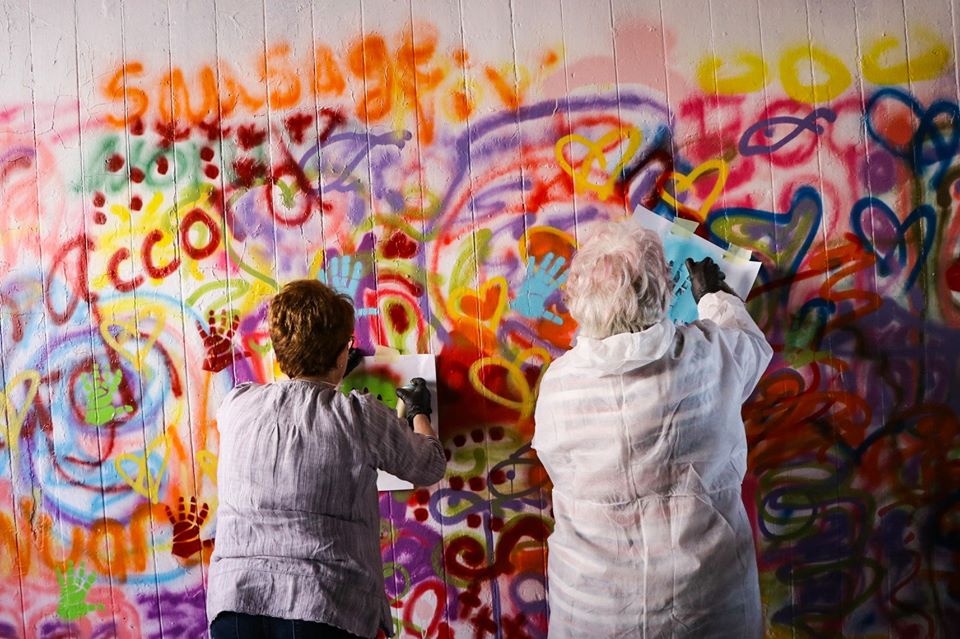In this landscape-oriented photograph, two older women are seen creating graffiti on a white slatted wall. Both women are wearing black latex gloves and various protective clothing: the woman on the left dons a purple blouse and has short brown hair with glasses, while the woman on the right, sporting short white hair, is clad in a white jacket. They stand facing the wall, holding stencils of handprints which they are spray-painting onto the surface. The wall itself is a vibrant canvas of colors and symbols, featuring orange spray-painted "Sausage" at the top left, "Accord" in red below it, multiple heart shapes in different colors, and a mix of other colorful swirls, lines, and dots. The lively and scattered graffiti includes various handprints, adding a psychedelic touch to the overall scene.